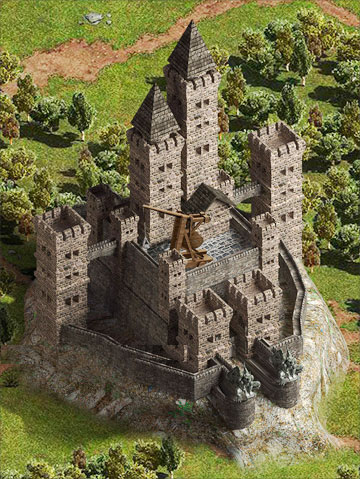The image portrays a grand, medieval castle constructed from beige stone, majestically situated on a rocky hill amidst lush, green grass and scattered trees. Captured from a high altitude—likely by a drone—the vertical photo highlights the castle’s intricate details. The structure features ten towers in total, including two prominent peaks with pointed, black slate, cone-shaped roofs at the rear, and two smaller, flat-topped columns at the front adorned with gargoyles. The castle is fortified by high walls and encircled by a robust gate. Two bridges extend from taller towers on the outskirts towards the main building. A notable feature is a catapult, reminiscent of ancient defenses, positioned conspicuously within the castle grounds.